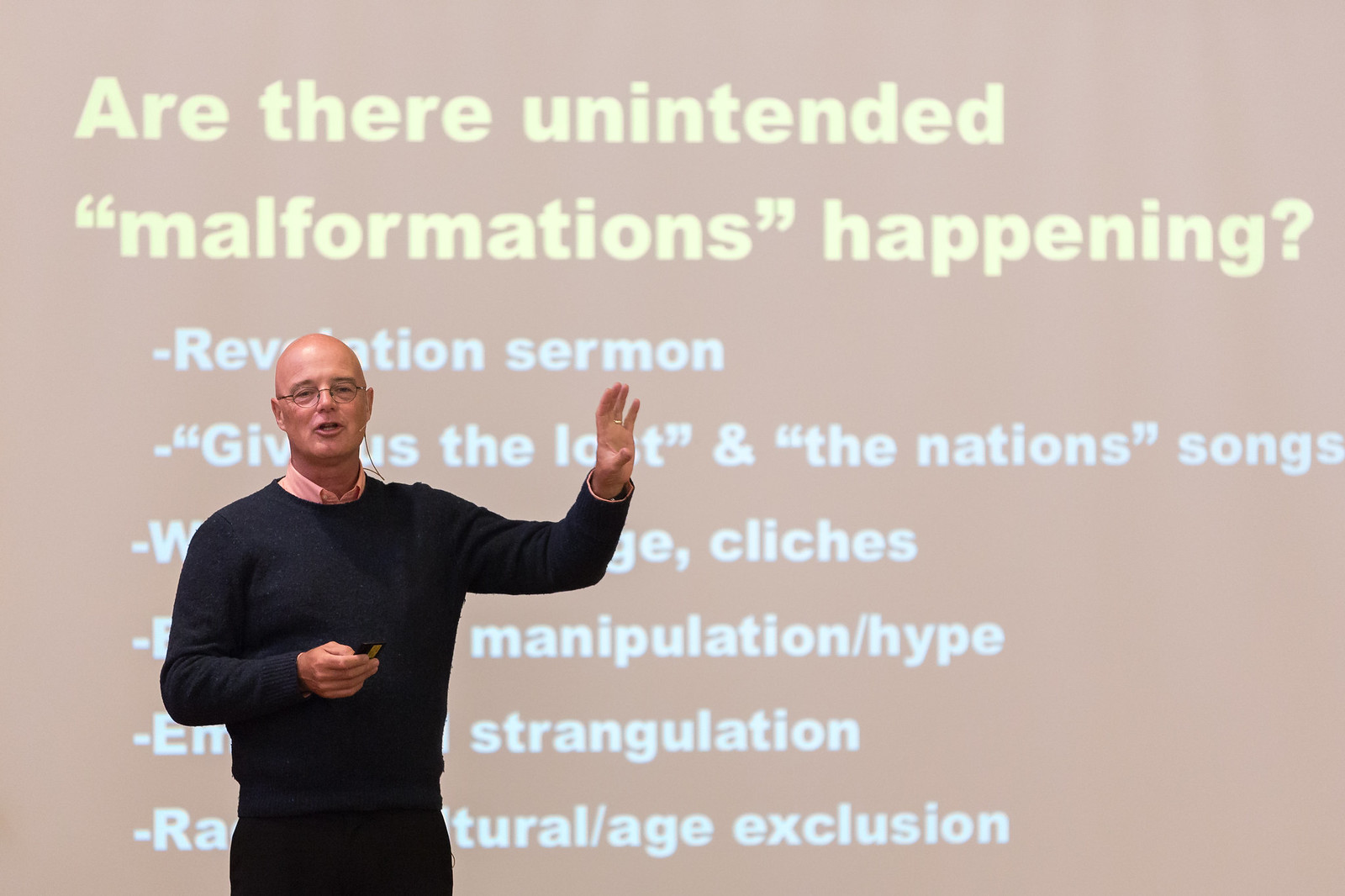In this image, a bald man with glasses is delivering a presentation. He is wearing a pink collared shirt under a dark blue sweater, paired with black dress pants. His left hand is raised in emphasis, while his right hand holds a remote clicker. A microphone is attached around his ear, indicating he is speaking to an audience, though they are not visible in the picture. Behind him, a projection screen features partially obscured text, including a title in yellow letters, "Are there unintended malformations happening?" Followed by phrases such as "revelation sermon," "songs," "cliches," "manipulation/hype," "strangulation," and "cultural age exclusion." The man stands in front of the text, partially blocking it with his body.